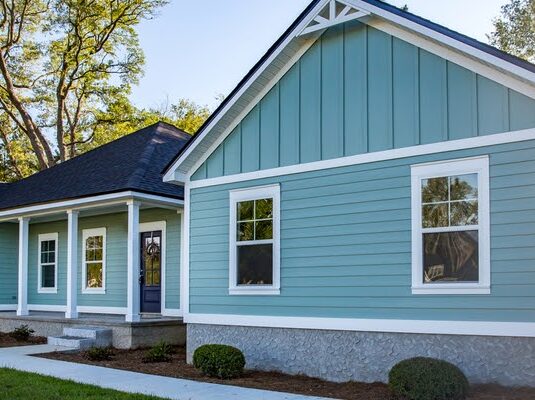This vibrant image captures the exterior of a connected, possibly dual-section home, characterized by its cohesive teal-blue siding and white trim. The house is slightly wider than it is tall, featuring a stone base that covers the bottom 10% of the structure. The left side resembles a welcoming front entrance, complete with a blue door on the right, two windows, and three vertical white pillars. A small raised porch with two steps leads up to this entrance, supported by three wooden posts.

The right side of the image hints at another part of the home, potentially a garage, which remains interconnected to the main structure, albeit with a noticeable gap suggesting a recessed connection. Both sections are topped with black roofs. 

The scene is set against a clear daytime sky, with lush green trees framing the upper corners of the photo. A paved walkway runs in front of the house, bordered by patches of soil and small plants, adding to the overall well-maintained and clean appearance of this blue home with its welcoming facade and inviting atmosphere.